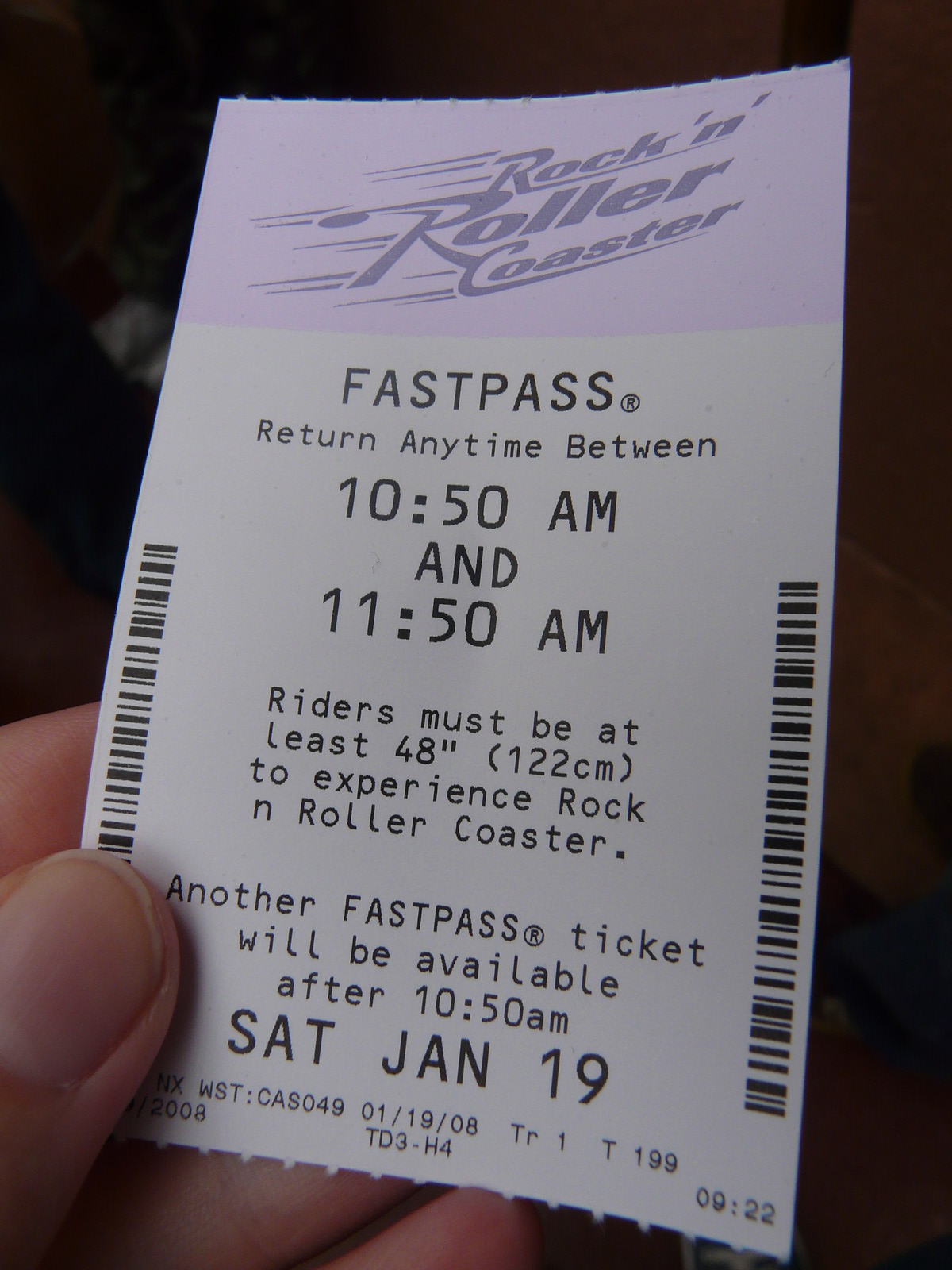In this rectangular image, a left hand with fair skin is holding a ticket against a mostly dark background with occasional lighter patches. The ticket, which is tilted diagonally to the right, has a light lavender rectangle at the top featuring the gray logo "Rockin' Roller Coaster" with an impression of motion. Black text on the white portion of the ticket states, "Fast Pass, return anytime between 10:50am and 11:50am." Additional details include the requirement for riders to be at least 48 inches (122 centimeters) tall, and a note that another Fast Pass ticket will be available after 10:50am on Saturday, January 19th. The thumb and partial fingers of the hand obscure the ticket's bottom left corner, where machine-readable barcodes and codes such as "terminal index WST: CAS049," the print date "01/19/08," and the time "09:22" are also present. The overall color scheme of the ticket features contrasting black and white tones.